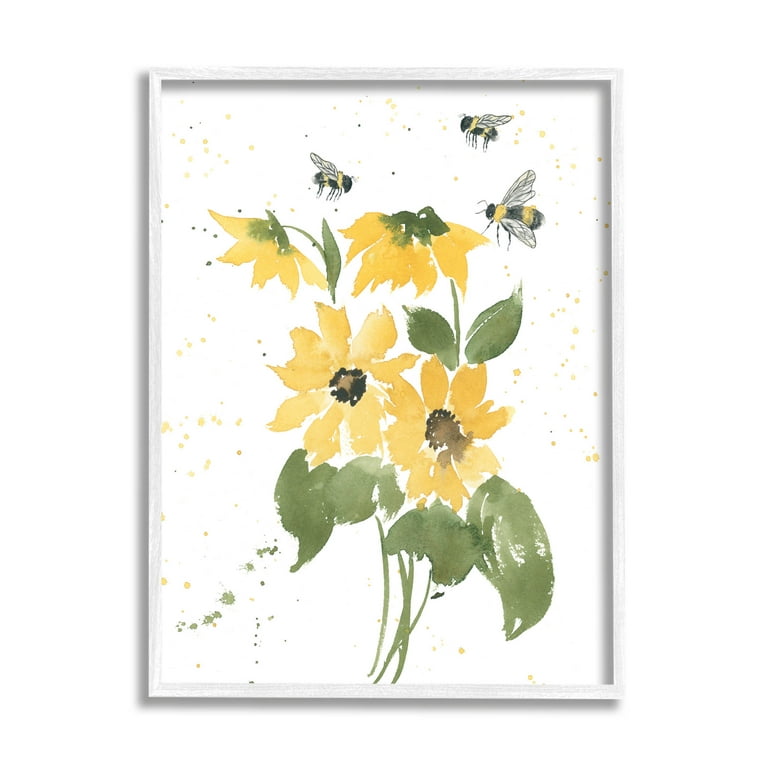This vertical rectangular artwork beautifully captures four yellow daisy-like flowers with dark centers, each supported by green stems and accompanied by large green leaves. The two lower flowers face forward, fully opened, while the two upper blooms bend downwards as if starting to wilt. Above these wilted flowers, three bees with black and yellow striped bodies and clear wings intricately detailed with black lines are seen in mid-flight, one bee heading to the right and the other two to the left, seemingly aiming towards the flowers. The background is predominantly white, embellished with numerous bright yellow and black spots that might represent pollen or possibly leaves being eaten by bugs. Framed elegantly within a narrow aluminum frame, this piece combines vivid colors and striking details, making the scene come alive.